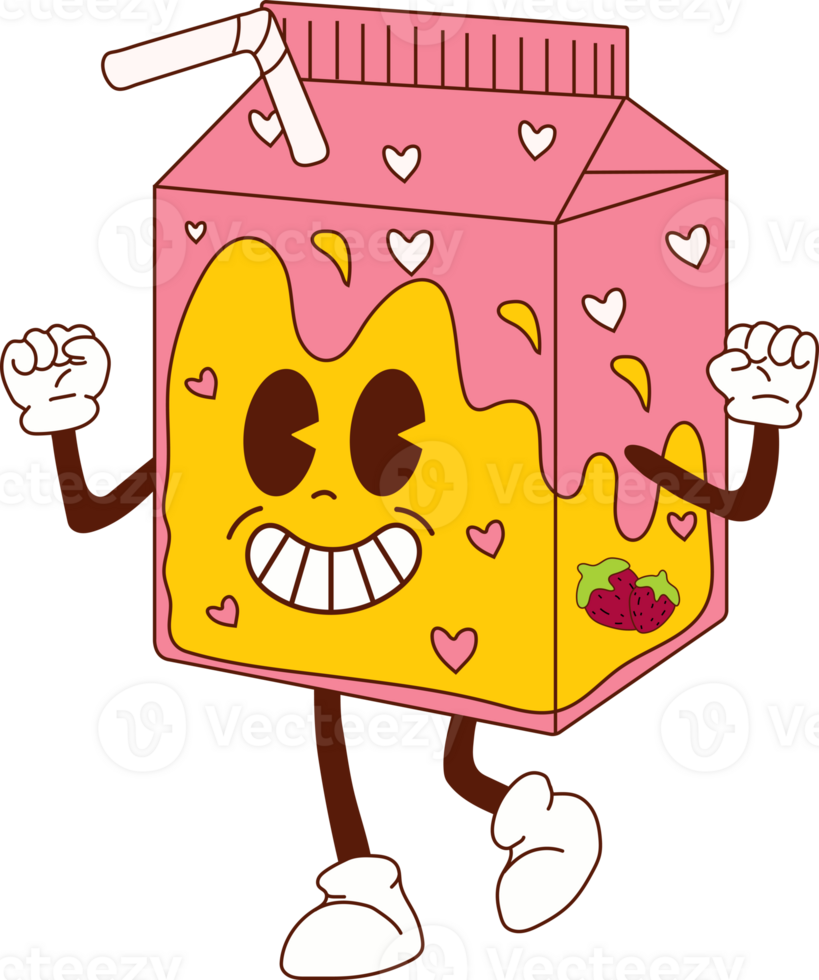This vibrant cartoon features a pink milk carton character set against a stark white background. The carton, designed to appear animated and lively, has a gabled top and a white straw protruding from the upper left side. It sports expressive, Pac-Man shaped brown eyes and a wide, toothy smile on a yellow face adorned with pink and white hearts. The box itself is decorated with delightful red strawberries with green stems and more white hearts with contrasting black outlines. The carton has two whimsical arms, ending in white gloves, and appears to be in motion, with one leg lifted and the other touching the ground. The arms and legs are drawn in black, with the legs ending in little white shoes. This charming and detailed rendering conjures a playful and cheerful character, reminiscent of familiar cartoon styles yet uniquely its own.